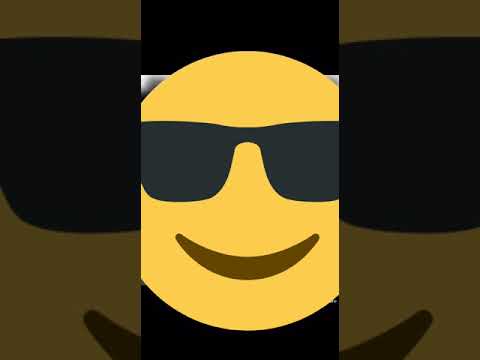The image features a central yellow smiley face emoticon wearing black, "cool dude" sunglasses and displaying a dark brown, upward-curved smile, all set against a black background. This central portrait is flanked by two vertical panels on the left and right, each showcasing a dimmer, semi-transparent, and fragmentary reflection of the smiley face. These panels mirror the left and right portions of the emoticon, with one highlighting the left sunglass lens and part of the smile, and the other doing the same for the right side. The design creates a split effect, visually dividing the frame into three sections, with the central smiley face as the focal point.